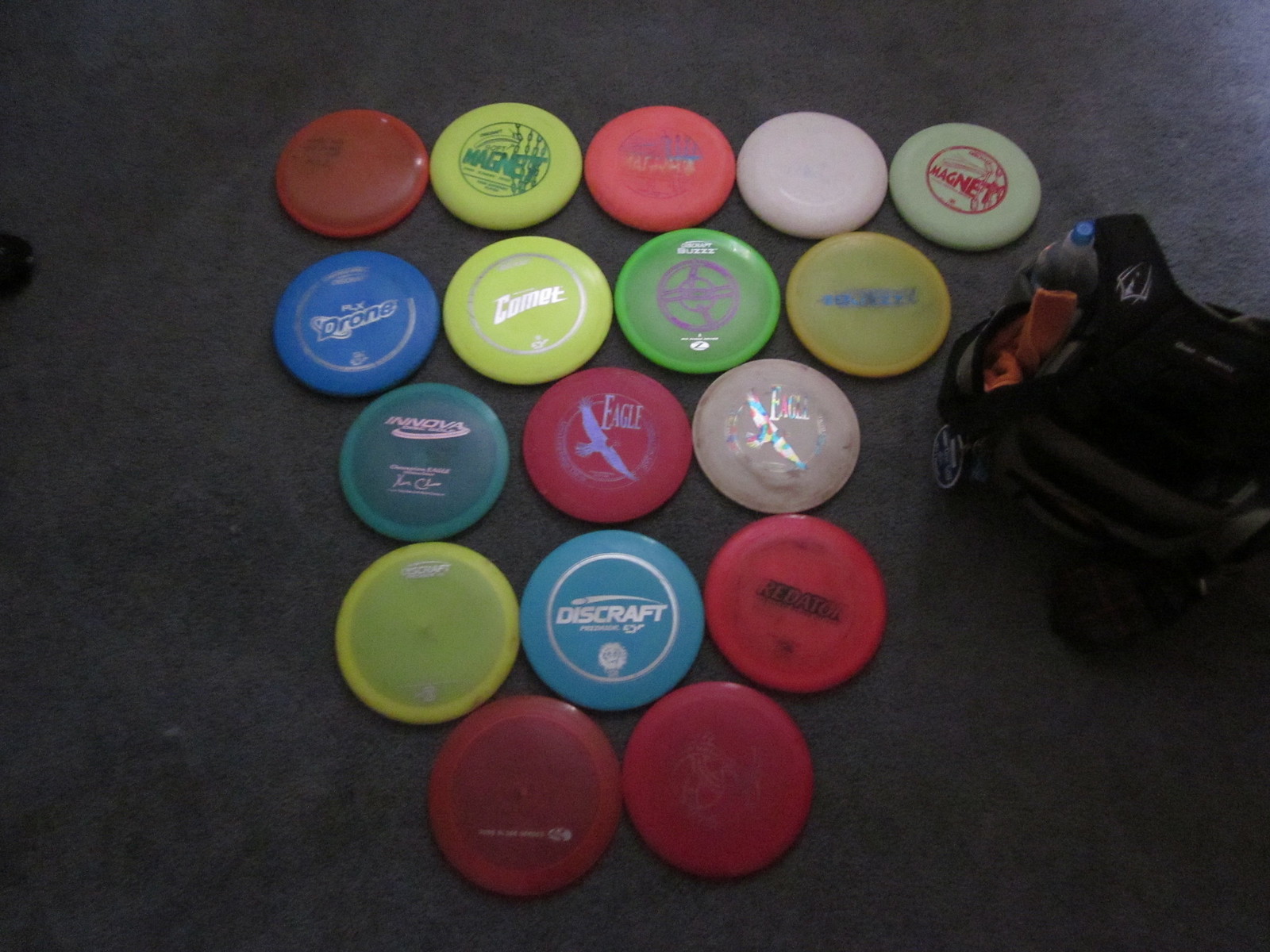This image captures an aerial view of a smoke gray concrete floor scattered with frisbees and a backpack. The dark gray backpack rests on the right side of the photo, featuring gray-trimmed pockets, a plastic water bottle with a blue cap, and a piece of orange paper sticking out. Centrally aligned are 17 neatly arranged frisbees in rows: 

- The top row has a red, yellow, pink, white, and light green frisbee.
- The row beneath has a blue, yellow, dark green, and light green frisbee.
- Next, there's an aqua, purple, and white frisbee.
- Following that, a yellow, light blue, and red frisbee.
- At the very bottom, two dark red frisbees can be seen.

Notable details include some frisbees with text such as "DISCRAFT" on a blue one with a white circle and another reading "MAGNET." The variety of colors spans from jelly orange, lime, hot pink, and teal, to unique designs like a rainbow pattern on aluminum foil.